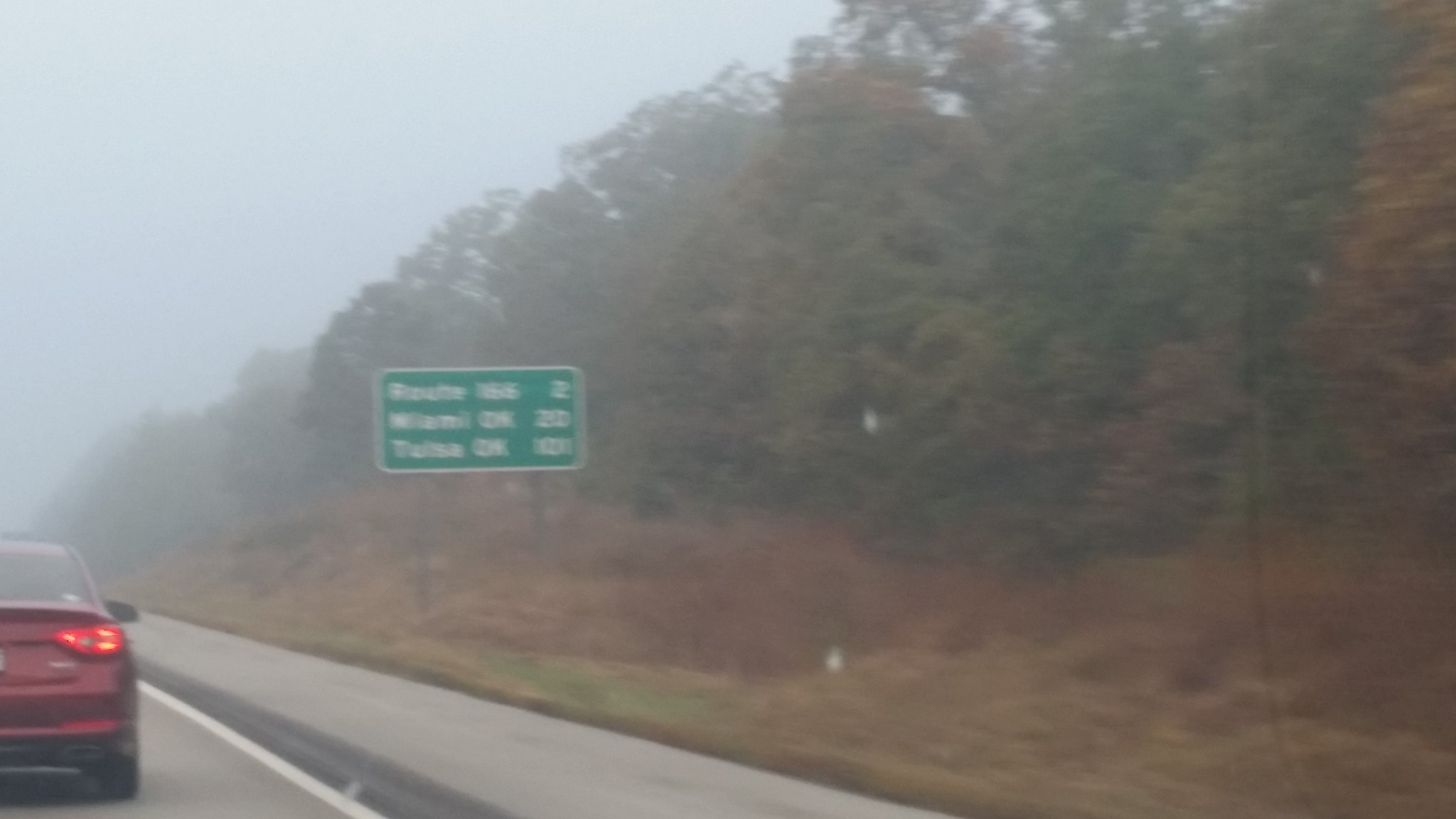The photograph, taken through the windshield of a moving car on a foggy day, captures the scene of an interstate highway. The image is notably out of focus, adding a mysterious haze to the surroundings. Dominating the left side is the rear of a maroon sedan with its brake lights illuminated. Directly in front, a standard green highway sign with white letters can be seen, though its details are blurred due to the motion and fog. The sign includes distances to several towns, with ‘Route 156’ possibly being 2 miles away, ‘Miami’ around 220 miles, and ‘Tulsa, Oklahoma’ approximately 210 miles away. On the right, a sidewalk can be partially noticed along with fall-colored trees and brownish-yellow grass lining the road, emphasizing the chilly, fog-laden atmosphere.